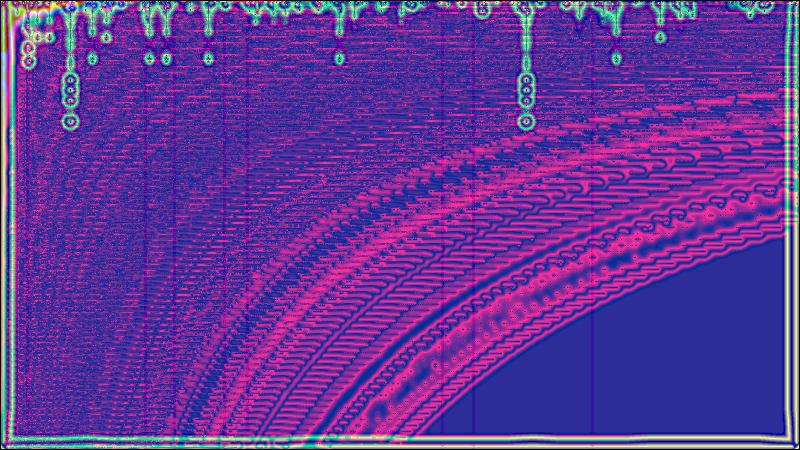The image is a color illustration in a modern, abstract style with a landscape orientation. The background is primarily a dark blue, accented by vibrant fuchsia textures that resemble tire tread marks, sweeping diagonally from the bottom right corner to the top left corner. This bottom right corner also features a solid purple arch from which the pink waves emanate and coalesce toward the upper left corner, where they lose definition and blend into a noise-like pattern. Across the top edge is a striking dripping effect of glowing green goo, some of which are hollow, with inner green dots, and depicted in varying lengths—some drips extending down nearly a third of the image. In the upper left corner, a subtle rainbow gradient overlaps with the green drips. Adding to the psychedelic and intricate nature of the graphic, a bright green rule forms a glowing border around the left, bottom, and right edges, encapsulating the entire composition.